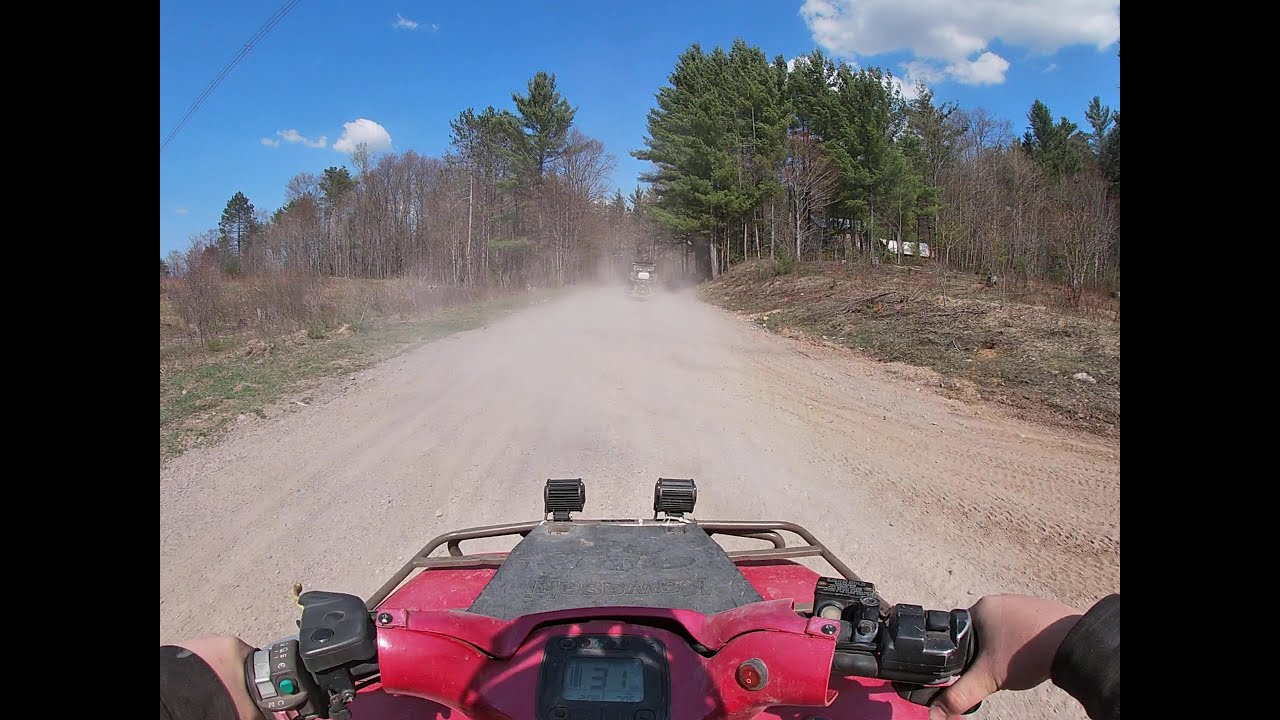The image captures the first-person perspective of a rider on a red ATV, framed by black borders on the left and right sides. The rider, wearing a black long-sleeve t-shirt, grips the handlebars firmly, with their right thumb visible. At the center of the handlebars, a digital display reads '33' and '1', likely indicating speed or other metrics. The scene ahead is dominated by a wide, dusty, and sandy-brown dirt road, with another vehicle visible in the distance, kicking up plumes of dirt. Flanking the road are patches of both dead and green grass, gradually giving way to several bushes and tall trees, some of which are barren, suggesting a fall setting. Overhead, the vibrant blue sky is dotted with light clouds, enhancing the sense of a clear, sunny day. Notable details include a green button on the left handle and a faintly discernible 'Kawasaki' logo on a small, dirty hood section of the ATV.